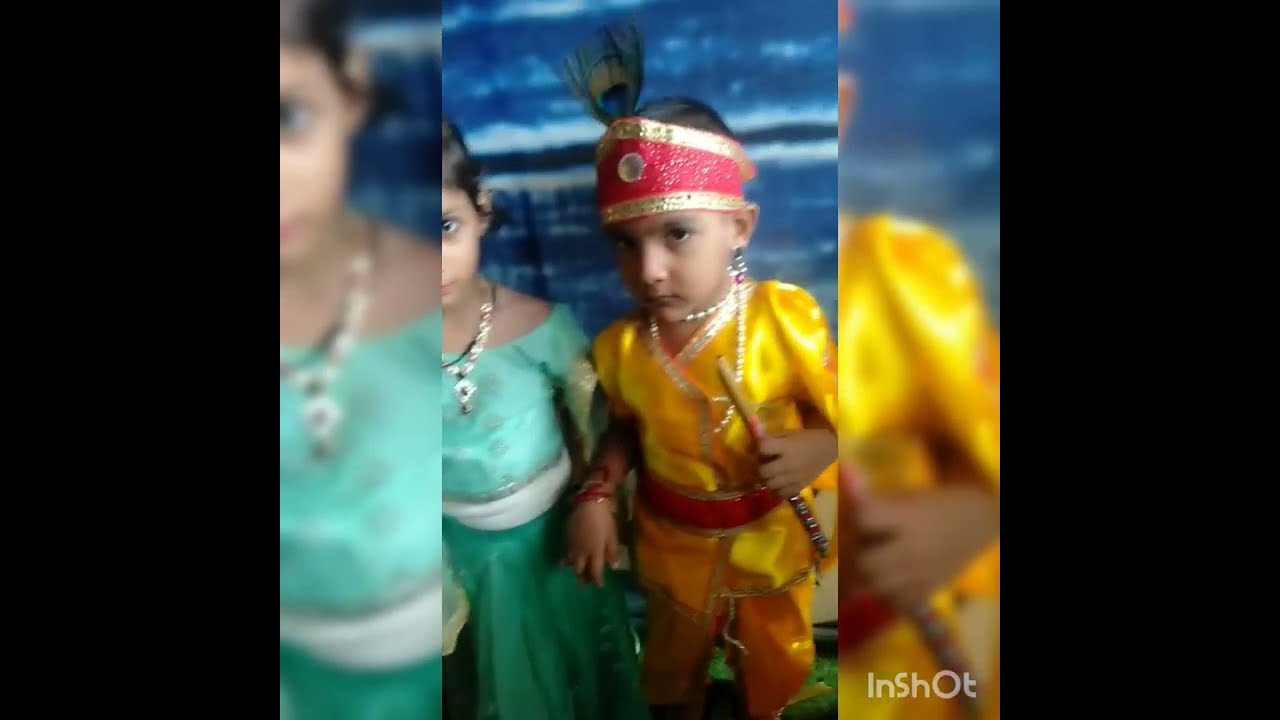This detailed photograph captures two young children standing side by side, evoking the essence of Princess Jasmine and Aladdin, likely dressed up for Halloween. The girl, positioned to the left, wears a striking long dress with a light turquoise bodice and a darker turquoise-teal skirt, complemented by a white sash around her waist and a prominent necklace. Her dark hair is neatly arranged, and her serious expression adds to the charm of her portrayal. Beside her, the boy dons a bright yellow satin outfit consisting of a top and pants, accessorized with a red belt around his waist and a red bracelet. He also sports a gold and red band around his forehead, complete with a peacock feather. He has dark hair and dark eyes, and like the girl, his expression is serious. In his left hand, he carries what appears to be a flute, enhancing his Aladdin-like appearance. The children hold hands between them, bringing a sense of unity to the image. The background is a mix of blue and white, and the photograph is framed with an intricate layout: blurred and enlarged portions to the immediate left and right, followed by a thick black border that encapsulates the entire scene.